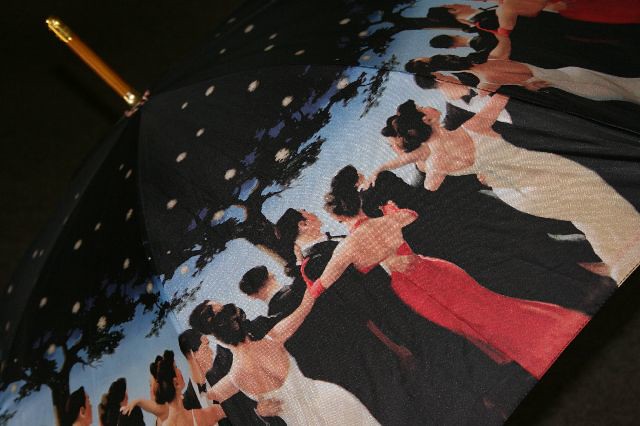This detailed photograph captures a unique, open umbrella set against a stark black background. The umbrella features a finely crafted wooden stick with a golden tip extending from the canopy's peak. The fabric of the umbrella is intricately decorated as if it were a canvas painting, depicting an elegant party scene. Within this scene, numerous people are engaged in dancing and festive activities. The men are dressed in black tuxedos and bowties, while the women are adorned in sophisticated evening gowns, predominantly in shades of white and red. The revelers are positioned facing away, seemingly gazing toward a large tree in the backdrop adorned with lights and ornaments. Dark green-leaved trees frame the scene, adding depth and contrast. Additionally, a pattern of white balls, resembling falling ornaments, cascades from the topmost part of the umbrella, enhancing its artistic allure.